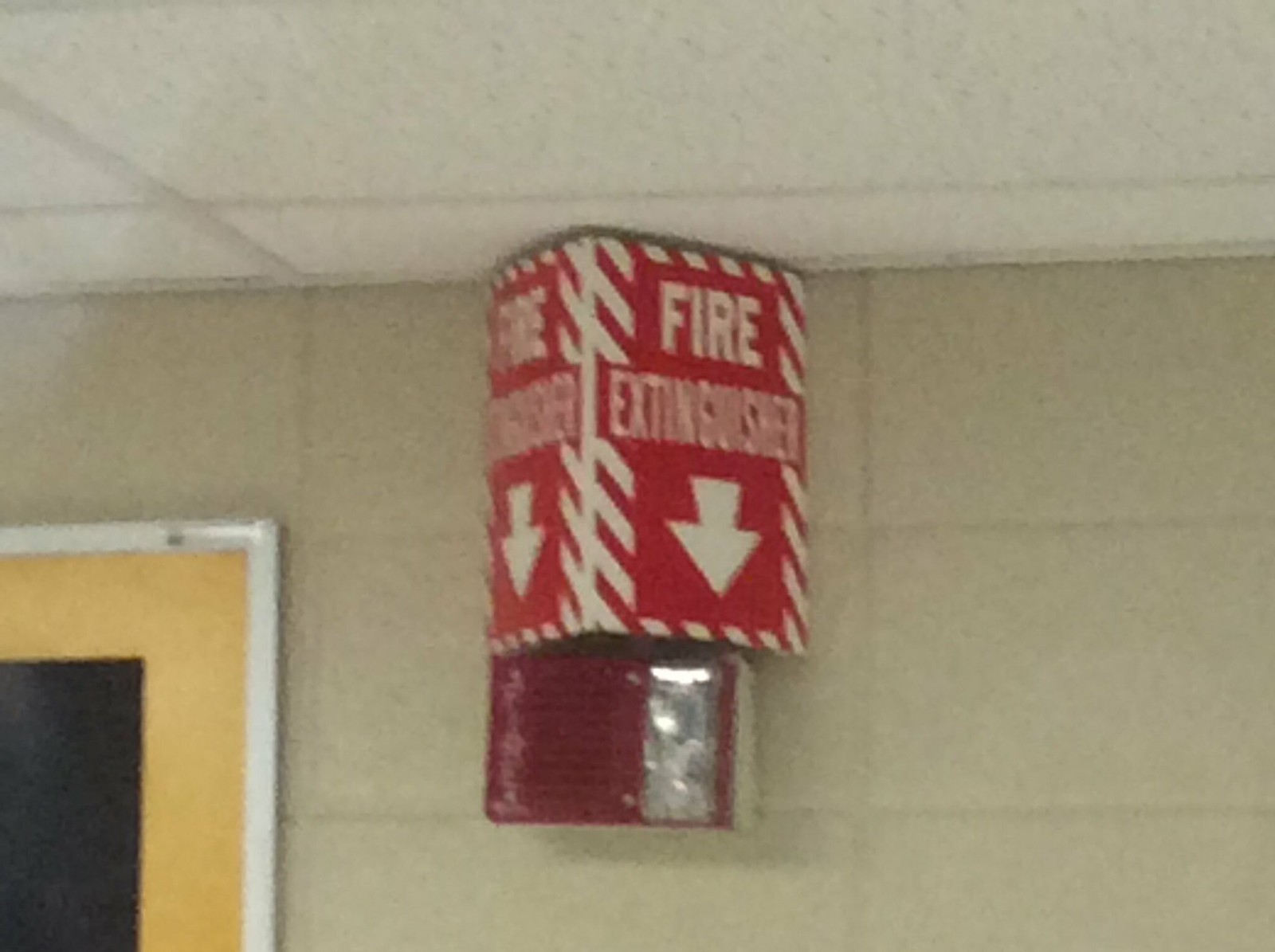In the out-of-focus and grainy photo taken in a hallway that resembles a school or another indoor building, several key details stand out. The hallway features a white drop ceiling with common ceiling tiles and cream or tan-colored brick walls. Prominently displayed in the center is a red and white fire extinguisher sign, marked with a downward-pointing white arrow and adorned with red and white stripes. This sign is visible from both sides, making it easily noticeable. Beneath the fire extinguisher sign, there's a square, dark red rectangular light with a white center, similar to a brake light, designed to flash brightly in the event of a fire. To the left of the sign and light, the edge of a door with a yellow hue and white trim is visible, potentially the framework for a classroom door. Altogether, the signage and light serve as crucial indicators for locating the fire extinguisher in an emergency.